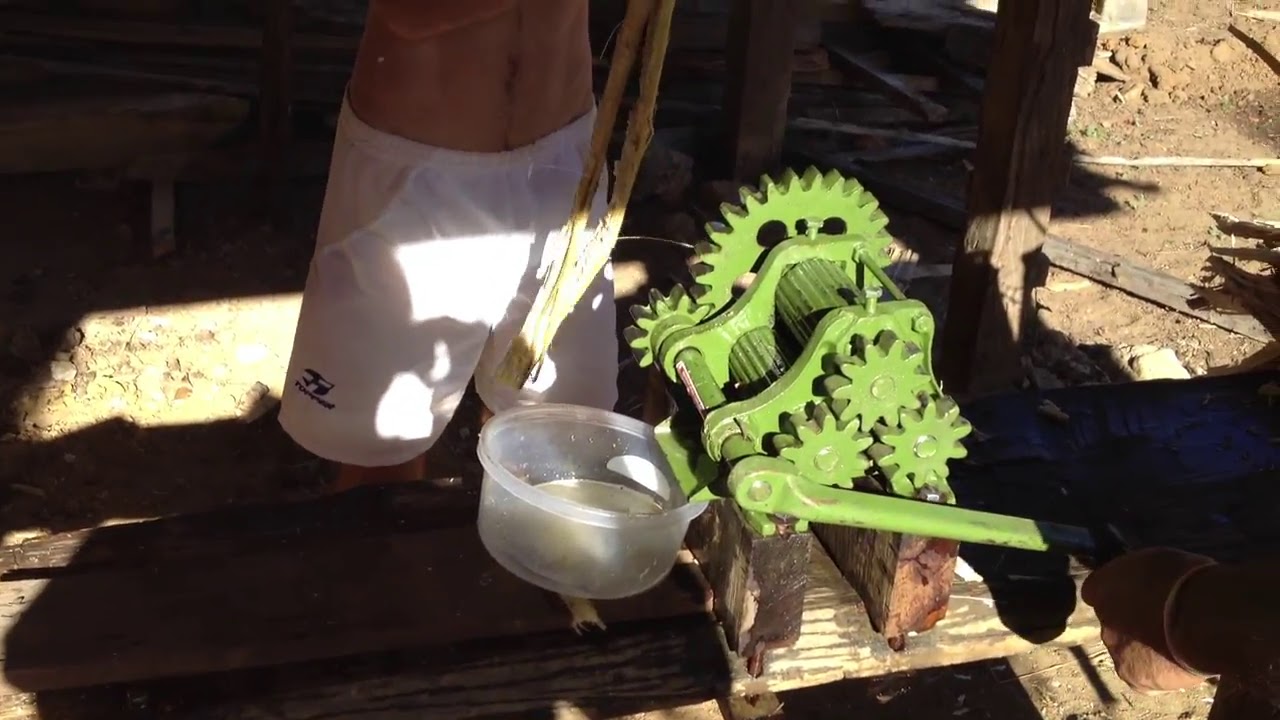This detailed color photograph, captured in landscape orientation, depicts an outdoor setting resembling an industrial work area or workshop, possibly near a shed, on a sunny day. Positioned in the top center of the image, slightly to the right, stands a shirtless man wearing white shorts. His partial view extends from his chest down to his knees, with his skin tone blending into the sunlight and shade of the environment.

Centrally featured in the image is an old, bright green hand-cranked machine mounted on a worn wooden plank. This machine, with its visible gears, rollers, and crank handle, appears to be some kind of press, possibly a juicer. A person's hand is seen operating the crank. In front of the machine rests a clear plastic Tupperware container collecting a white liquid, hinting at the machine's function.

Surrounding the main elements are various scattered wood planks and a dirt-covered ground, adding to the rugged, makeshift ambiance of the scene. The color palette features different shades of brown, green, white, black, and touches of orange, enhancing the realism and representational style of the photograph.